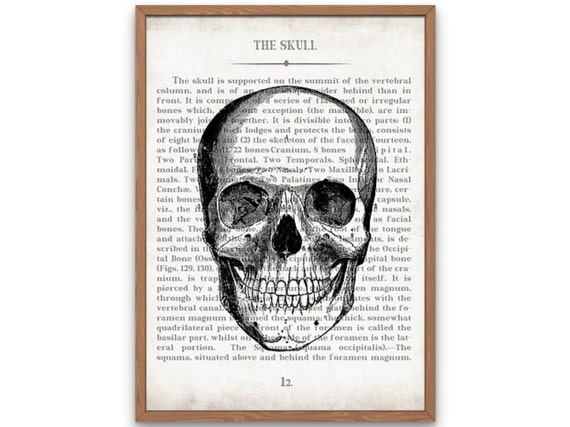The image features a framed portrait-oriented poster with a light wooden frame. The background of the poster resembles aged white paper, creating a vintage feel. At the top of the poster, the bold headline reads "The Skull," followed by a vertical line. The text, justified on both the right and left, describes the anatomy of a human skull, starting with the phrase, "The skull is supported on the summit of the vertebral column."

Printed over the text is a detailed black ink illustration of a human skull, facing the viewer. The illustration includes shadowing around the eye sockets and nasal cavity, producing a three-dimensional effect. Additional text towards the bottom of the page includes page number "12" and mentions anatomical details, though some parts are partially obscured by the illustration. The framed poster appears to float against a clean white background common in representational-style photographic setups.